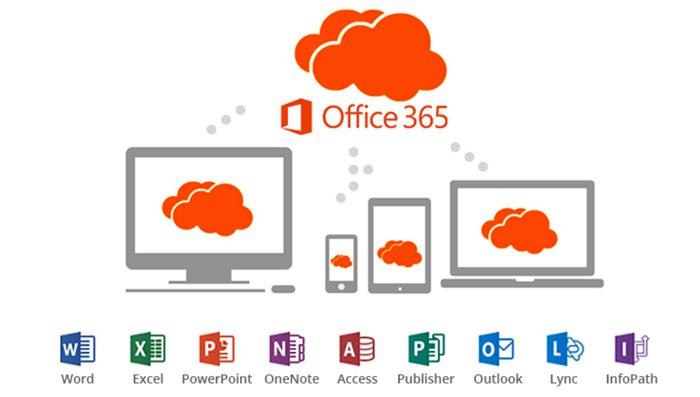The image is a digitally produced graphic displayed on a screen. At the top of the picture, there are two orange clouds. Directly beneath these clouds, in orange text, is the label "Office 365" enclosed within a three-dimensional square box. Dotted lines extend downward from the clouds, connecting to a series of electronic devices arranged from left to right: a computer, a smartphone, a tablet, and a laptop. Each device displays the same orange clouds on its screen, with the image sized proportionately to fit the smaller screen of the smartphone.

Below the devices, there is a row of clickable icons resembling open books or envelopes. These icons represent various Microsoft Office applications. From left to right, the icons include:

1. **Word** - Represented by a blue book with a white "W."
2. **Excel** - Depicted as a green book with a white "X."
3. **PowerPoint** - Shown as a red book.
4. **OneNote** - Displayed as a purple book.
5. **Access** - Appearing as a red book.
6. **Publisher** - Illustrated as a blue book.
7. **Outlook** - Represented with an icon.
8. **Lync** - Another specific icon.
9. **InfoPath** - Displayed as a purple book.

The colors and icons visually distinguish each application, making it easy to identify and click on them.